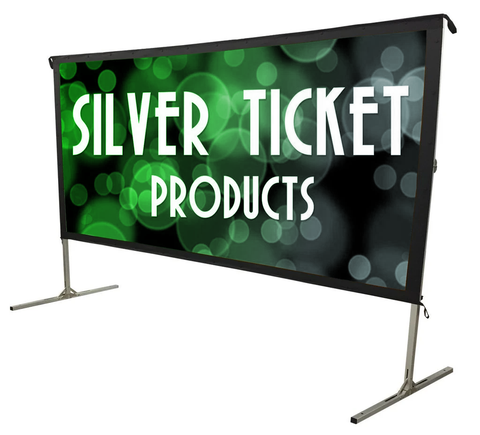The image features a rectangular projection screen or net-like structure held up by two metal poles, each extending into horizontal feet anchored to the ground on both sides. The screen is depicted at an angle, with the left side appearing further back than the right. The background is a solid white, emphasizing the digital nature of the composition, likely created using Photoshop or similar software. The screen has a black border with black hooks or tags visible on the top left, top right, and bottom right corners. In the center of the screen, bold white text reads "Silver Ticket Products" across two lines. The screen's background is filled with floating green and blue bubbles against a black backdrop, resembling sunspots or light distortions captured by a camera. The product display suggests it’s a digital markup of an actual net-like projection screen.